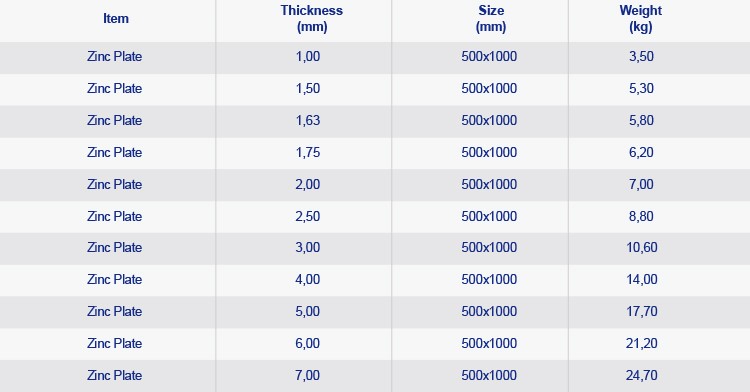This image depicts a detailed chart related to zinc plating, displaying various material specifications organized by item, thickness, size, and weight. The chart, differentiated by light gray and dark gray shades, features blue-font text. Each item is labeled as a "zinc plate." The thickness column, measured in millimeters, lists increments from 1.00 mm to 7.00 mm. Despite the size remaining consistent at 500 mm by 1000 mm across all entries, the weight column, measured in kilograms, varies significantly, ranging from 3.50 kg to 24.70 kg. This visual representation effectively highlights how the weight of zinc plates increases with thickness while maintaining the same dimensions.